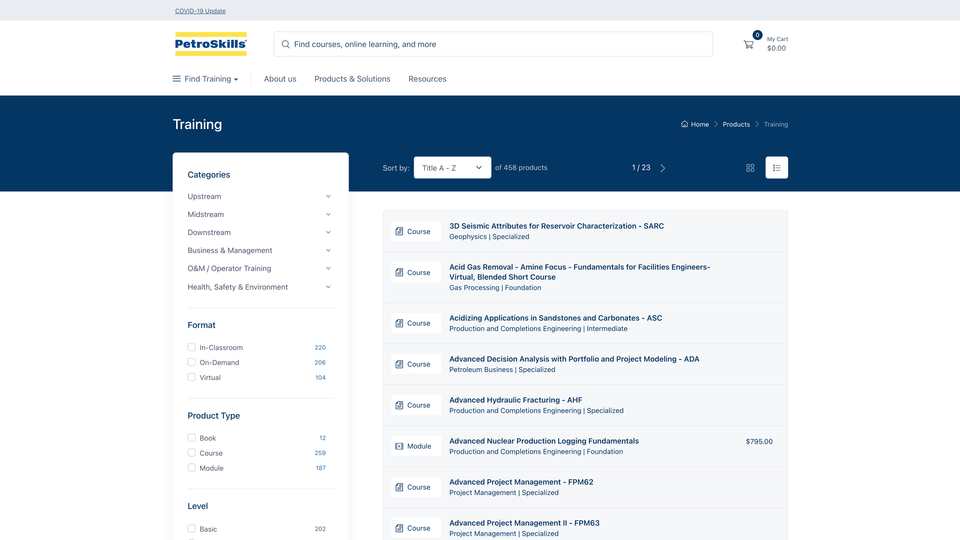At the top of the image, there is a long blue strip containing some text in blue print. Below this strip is a long white box with blue text that reads "Petrol Skills," framed by yellow lines above and below it. To the right of this, there is a search box with the placeholder text "Find Courses, Online Learning, and more," accompanied by an icon of a shopping cart. The cart has a blue circle with the number three inside it, indicating three items, along with a total price display.

Adjacent to these elements is a navigation section comprising three horizontal lines labeled "Find Training," as well as a drop-down menu containing options like "About Us," "Solutions," and "Resources." Below this is a large dark blue box labeled "Training," which features sorting options. A text block shows "Sort By," and there is a small box labeled "A to Z of 458 products," with pagination controls showing "1 of 23" and a right arrow next to it.

Underneath the sorting area, a light blue box contains further navigational aids, including a drop-down menu to filter by "Categories," "Formats," "Product Type," and "Level."

On the right side of this layout is a large blue section showcasing different courses, each listed in blue text. Every course entry includes a small white button labeled "Course" next to the course title. Notably, the third course from the bottom is priced at $795.